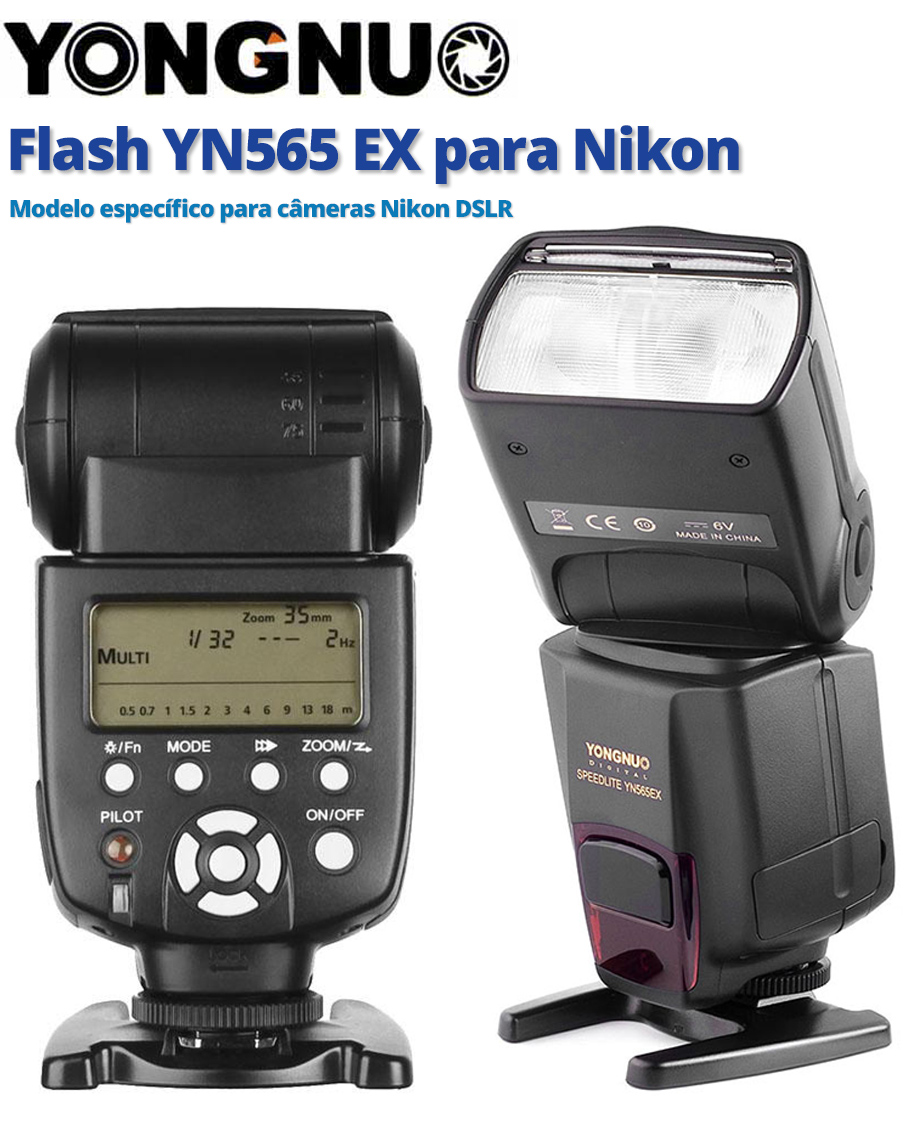This is an advertisement for a DSLR camera accessory, specifically a Yongnuo Flash YN-565EX designed for Nikon cameras. The upper left-hand corner of the image contains the branding and model information: "Yongnuo" in black text and "Flash YN-565EX Para Nikon" in dark blue text. Below that, light blue text reads "Modelo Especifico Para Camaraz Nikon DSLR." The product is shown from two angles: the back view displays a digital display with several white buttons for functions such as mode, zoom, and system navigation, all housed in a black plastic base. The front view reveals a rectangular-shaped white light or sensor, with the bottom half featuring a clear red trapezoidal button area.